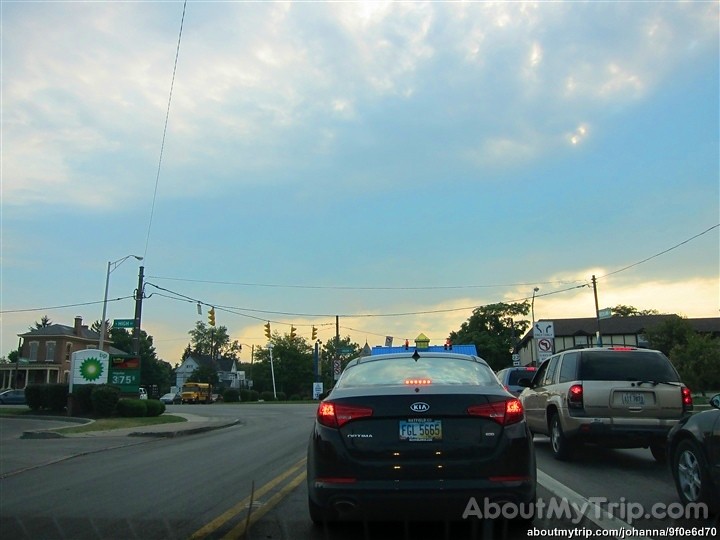The image, captured from a dash cam mounted on the front of a car, depicts a scene at a four-way intersection. The vehicle is halted at a red light, as indicated by the red traffic signal directly ahead. To the right, a line of cars is visible, also waiting at the light, while the left-hand lane is completely devoid of vehicles. Prominently on the left side of the image is a BP gas station, easily identifiable by its distinctive green and yellow sunburst logo. Traffic lights are suspended on lines strung across the intersection, with signals facing in all four cardinal directions: north, south, east, and west. Additional traffic signs are visible, including indications prohibiting right and left turns from the lane the car is in, suggesting that the only permissible direction for travel is straight ahead.